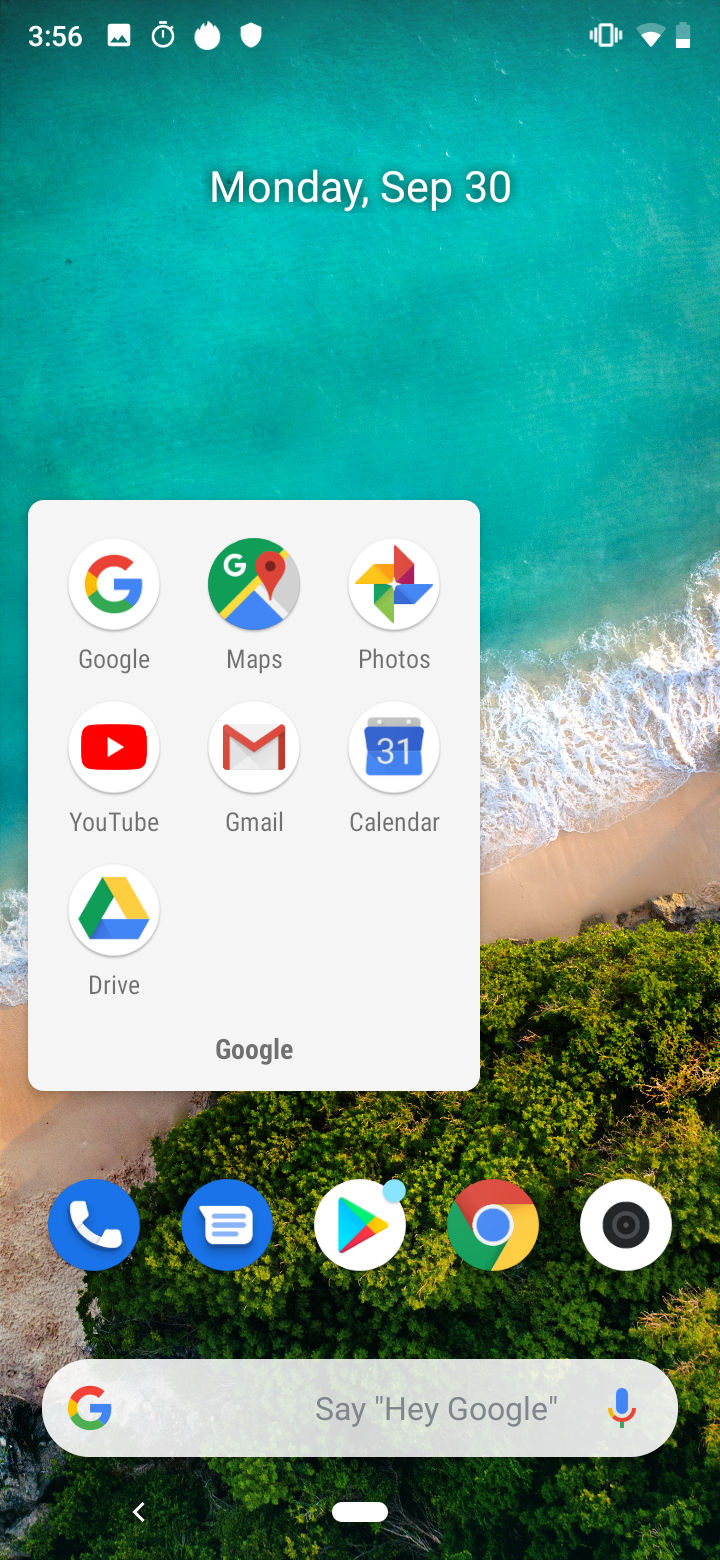**Detailed Caption**: The image showcases the front screen of a smartphone categorized under Websites. The phone displays a visually appealing beach-themed wallpaper with vivid blue water, rolling white waves, sandy shores, patches of lush greenery, and scattered rocks. The screen indicates that 356 pictures have been opened and it is Monday, September 30th. 

At the top-right corner, the status icons reveal that the phone is on vibrate mode, the battery is nearly depleted, and it's connected to Wi-Fi. 

The primary focus is a folder labeled "Google" containing several apps: Google, Maps, Photos, YouTube, Gmail, and Calendar. Positioned just below this folder are the navigation bar icons, which include the phone dialer icon, messaging icon, Play Store icon, Chrome browser icon, and a camera icon that resembles a camera lens.

At the bottom of the screen, there is a Google search bar with a microphone icon and the prompt "Hey Google," flanked by the Google logo. The arrangement on the screen is straightforward, with a clean, organized layout, emphasizing functionality and ease of access to essential applications.